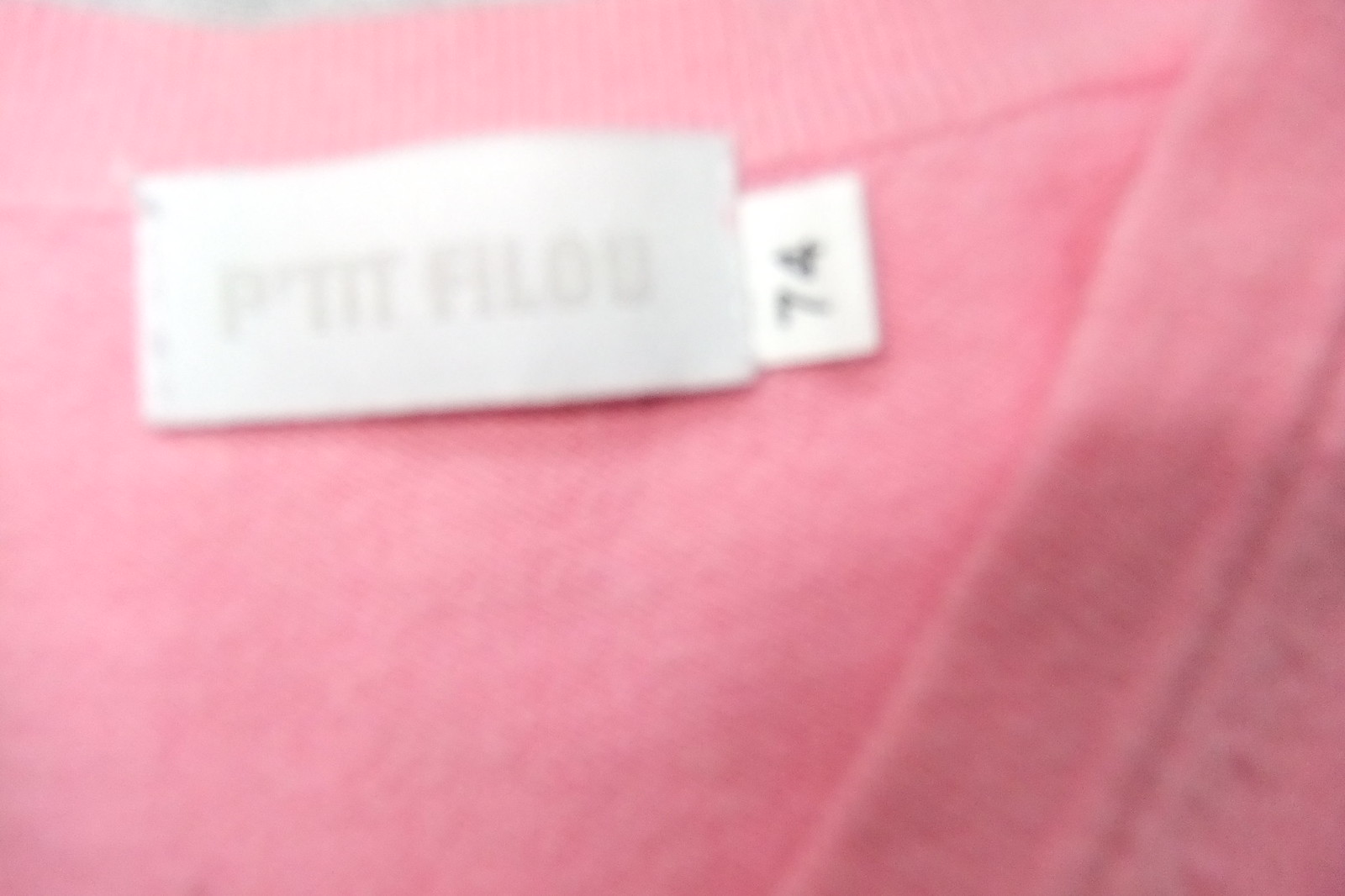This image captures a close-up view of the back collar area of a V-neck shirt, showcasing the intricate texture of its fabric. The material appears to be a blend, likely consisting of around 50% cotton mixed with another fabric, possibly silk, giving it a soft yet structured appearance. The focal point of the image is the white tag situated at the center of the V-neck collar, complemented by a smaller adjacent tag that reads "74". The shirt itself is a soft pink color, with the brand name "P-T-I-T-F-I-L-O-U" faintly printed in a light white hue on the main tag, although the letters are somewhat difficult to discern due to their subtle color contrast against the tag’s background. The V-neck design is clearly visible, with the collar dipping diagonally down rather than forming a circular or crew neckline.